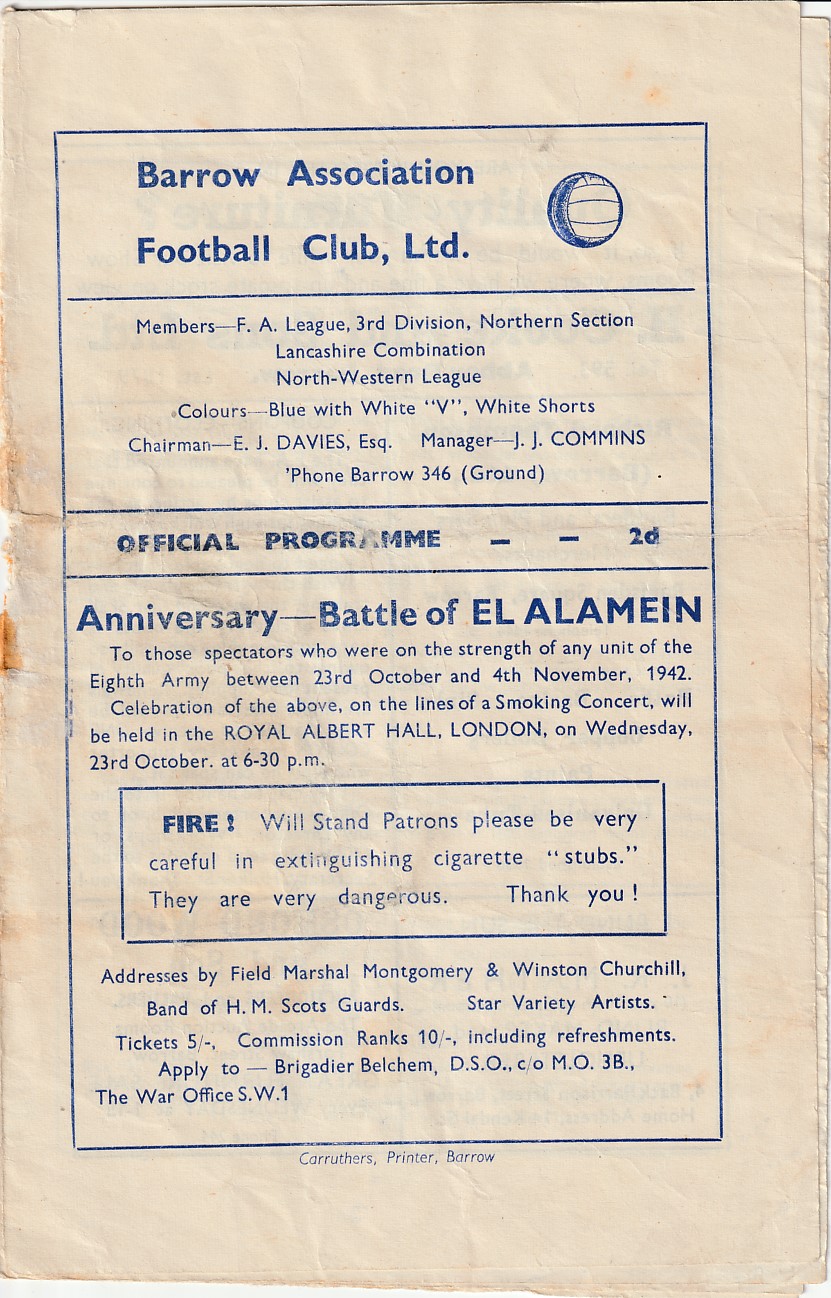This image is a vintage page from an official program or magazine, likely for a football club, featuring aged, wrinkled white paper reminiscent of parchment. The text is enclosed in a blue rectangular border and printed in blue font. At the top, it reads "Barrel Association, Football Club Limited," accompanied by a logo featuring a round football. The program details the club's affiliations, listing "Members, F.A. League 3rd Division Northern Section, Lancashire Combination, Northwestern League", and notes the team colors as "blue with white V, white shorts." It also provides key officials: Chairman E.J. Davies Esquire and Manager J.J. Commons, along with the phone number "Barrel 346" and mentions the ground. It is identified as an "Official Program, 2D," and commemorates the "Anniversary Battle of El Alamein." Additional warnings urge "spectators who are on the strength" to extinguish cigarette stubs carefully to prevent fires. The overall aesthetic shows signs of age with a patina turning the paper into a yellowish-beige hue, preserving the historic essence of the event it represents.